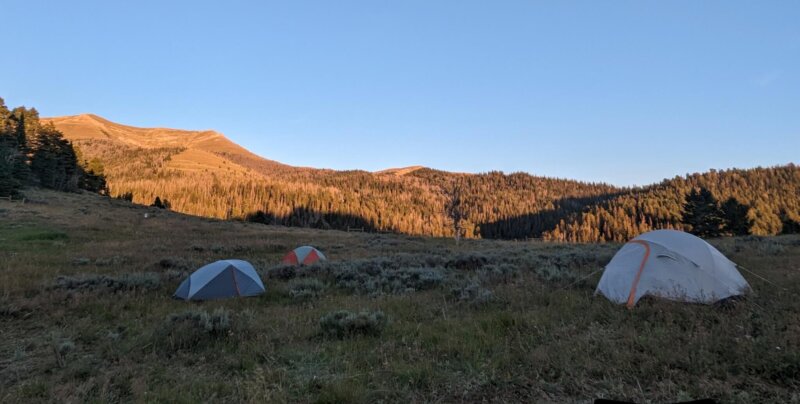This serene photograph captures a picturesque camping scene at sunrise. Three pop-up tents are scattered across a green, grassy meadow, creating a peaceful ambiance. The foreground features a white tent with a yellow door on the right, and two smaller tents to the left—one orange and white, and the other gray and white with a triangular pattern. The meadow, still shaded and dark from the early morning light, contrasts beautifully with the surrounding landscape. 

In the background, a majestic mountain range basked in golden sunlight rises up, partially covered in a mix of green and brown trees, evoking a forested feeling. The hills exhibit lighter brown hues, and a grove of pine trees is visible to the left. Above, the sky is a perfect light blue, almost entirely cloudless, adding to the tranquil beauty of the scene. The golden illumination on the mountains suggests the sun has just risen, enhancing the peaceful and refreshing atmosphere of this natural setting.